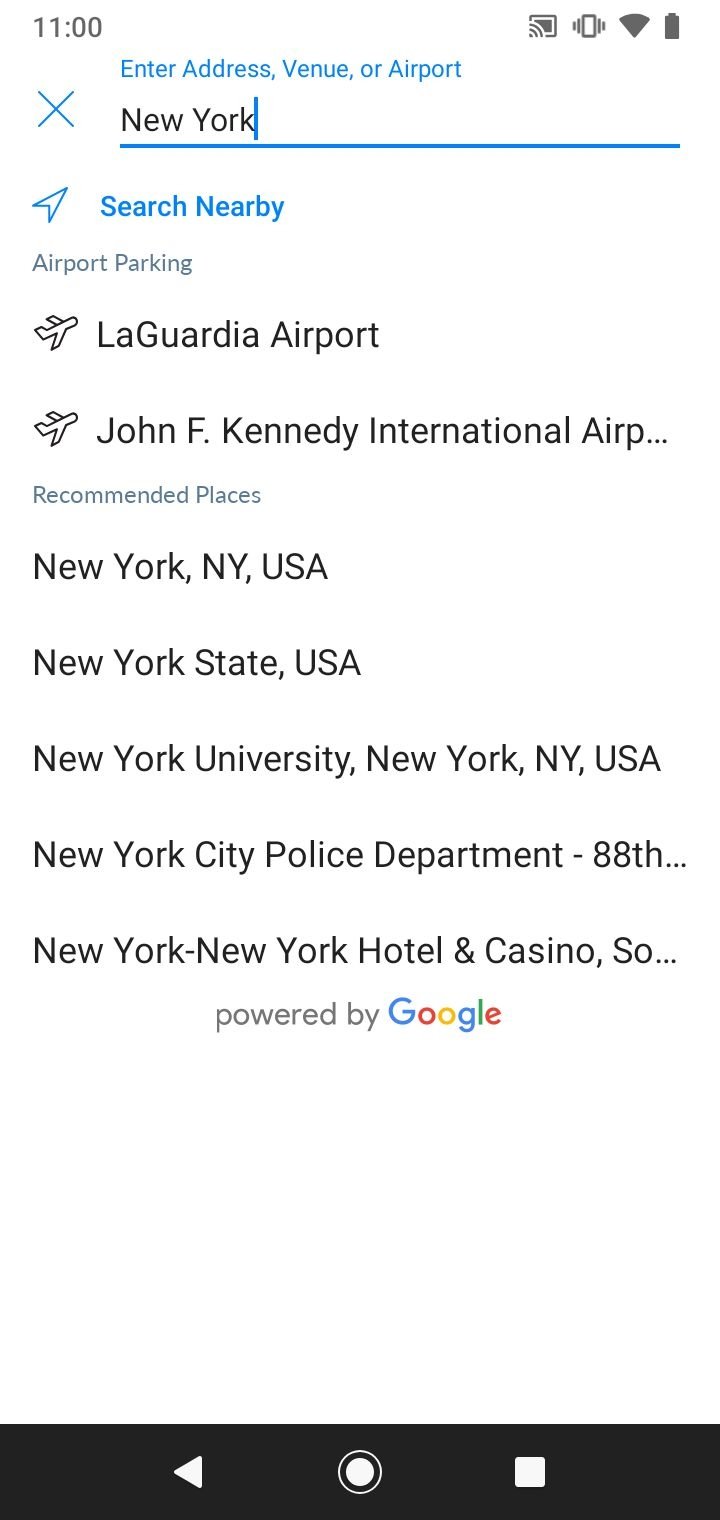At the very top left corner of the page, the number "11" is displayed. Moving across from left to right, various icons are visible, including representations for the internet and battery, with two additional, unidentified icons preceding them. Beneath the number "11," the text "Inter-address, View, or Airport" is written, followed by a prominent blue "X" and a blue line. Below this blue line, the word "New York" is printed in bold black letters. Directly under "New York," there is a sideways triangle arrow icon accompanied by the text "Search Nearby."

Further down, under the “Airport” category, there is a small airplane icon next to the name "LaGuardia Airport" and another airplane icon preceding the name "John F. Kennedy International Airport." Underneath these, the section titled "Recommended Places" lists several entries: 
1. New York, New York, USA
2. New York State, USA
3. New York University
4. New York, New York, USA again
5. New York City Police Department 88th Precinct
6. New York, New York Hotel and Casino

Following the list of recommended places, the phrase "Powered by Google" appears in smaller text, with the word "Google" displayed in its signature multi-colored logo, while all other text is in black.